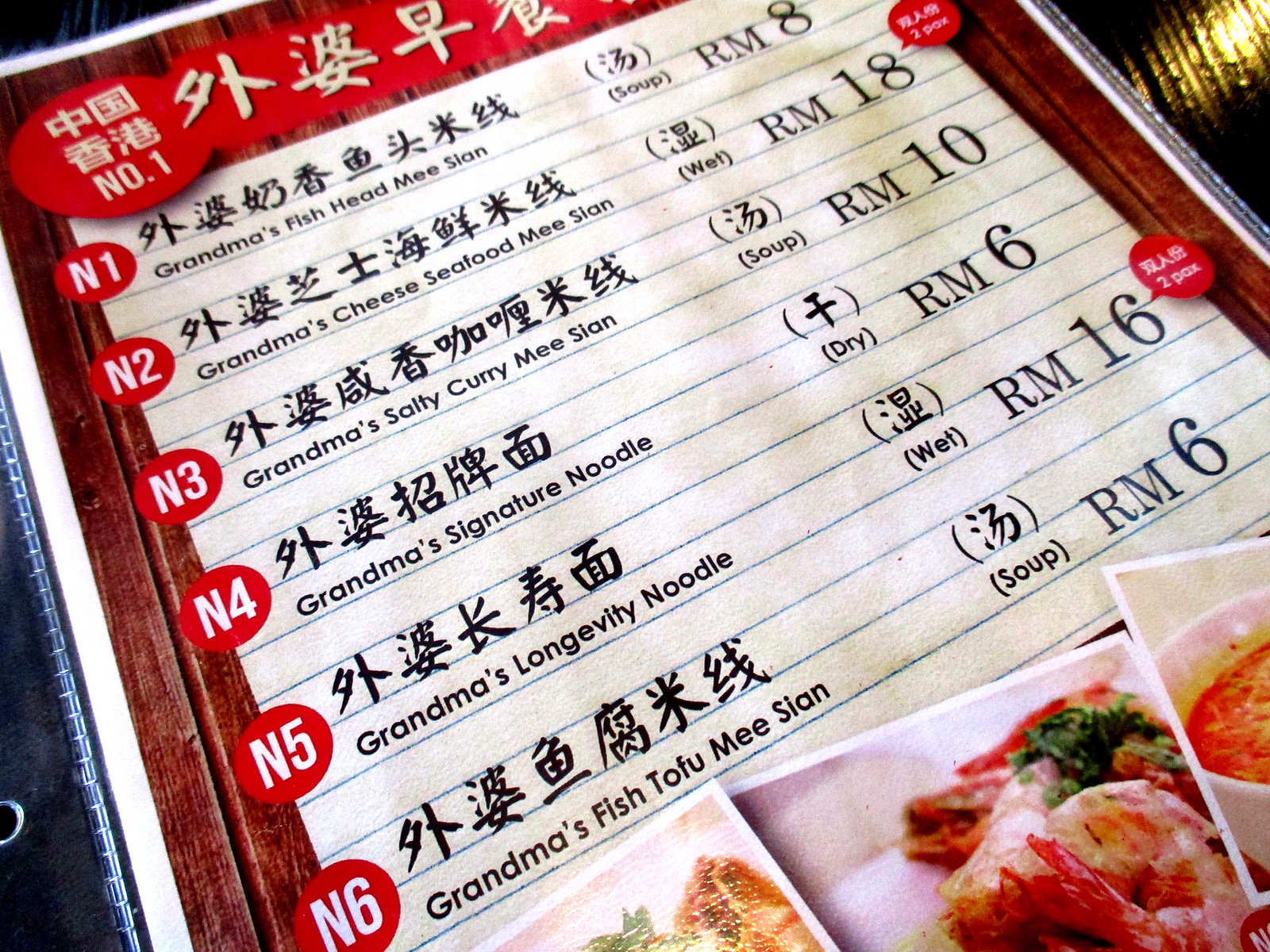This photograph depicts a slightly tilted menu card from a restaurant, written in both English and Chinese. The menu card is divided into a left-hand column listing six dish names, each prefixed with "N" and a number (N1 to N6), and a right-hand column indicating the type and price of each dish. 

The dishes listed are:
- N1: Grandma's Fish Head Mie Sian, Soup - RM 8
- N2: Grandma's Cheese Seafood Mie Sian, Wet - RM 18
- N3: Grandma's Salty Curry Mie Sian, Soup - RM 10
- N4: Grandma's Signature Noodle, Dry - RM 6
- N5: Grandma's Longevity Noodle, Wet - RM 16
- N6: Grandma's Fish Tofu Mie Sian, Soup - RM 6

The menu is protected by a plastic cover and bordered with a white edge and a brown border that resembles wood. At the top of the menu card, there is a partially visible red section adorned with white symbols, one of which is the number "1." Vertically listed along the left side are red circles marked with N1 to N6, each followed by the dish name in English and Chinese characters. On the right-hand side, each dish type (soup, wet, dry) and the corresponding price are listed in black text.

The bottom of the menu features partial images of the dishes, and a bit of the black surface on which the menu rests is visible in the lower left-hand corner.